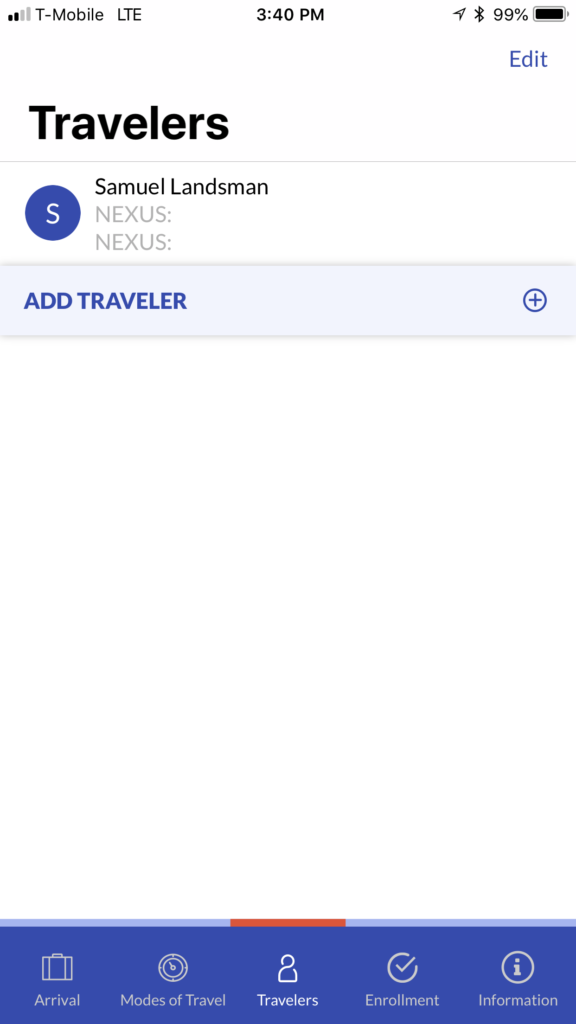This screenshot showcases a travel management page, seemingly from a service like Southwest Airlines, as suggested by the color scheme. The top of the image displays status information including "T-Mobile LTE," the time "3:40 PM," and a battery indicator at 99%. Below this, the main section of the page lists travelers. The first traveler is identified as Samuel Landsman, with his name enclosed in a blue box labeled "S." Listed beneath Samuel's name is the repeated word "Nexus."

A prominent feature on the page is a blue box with the text "Add Traveler" in blue font, accompanied by a blue plus sign enclosed in a circle, allowing users to add more travelers to the itinerary. The remainder of the screen features a white background.

At the bottom, a blue navigation bar contains five options. The icons and labels for these options are:
1. Arrival, represented by a briefcase,
2. Modes of Travel, depicted with a tire,
3. Travelers, indicated by a small person icon,
4. Enrollment, denoted with a checkmark,
5. Information, symbolized by an "i".

Each option provides a different function pertaining to travel management and traveler information, but specific flight details are not displayed on this page.